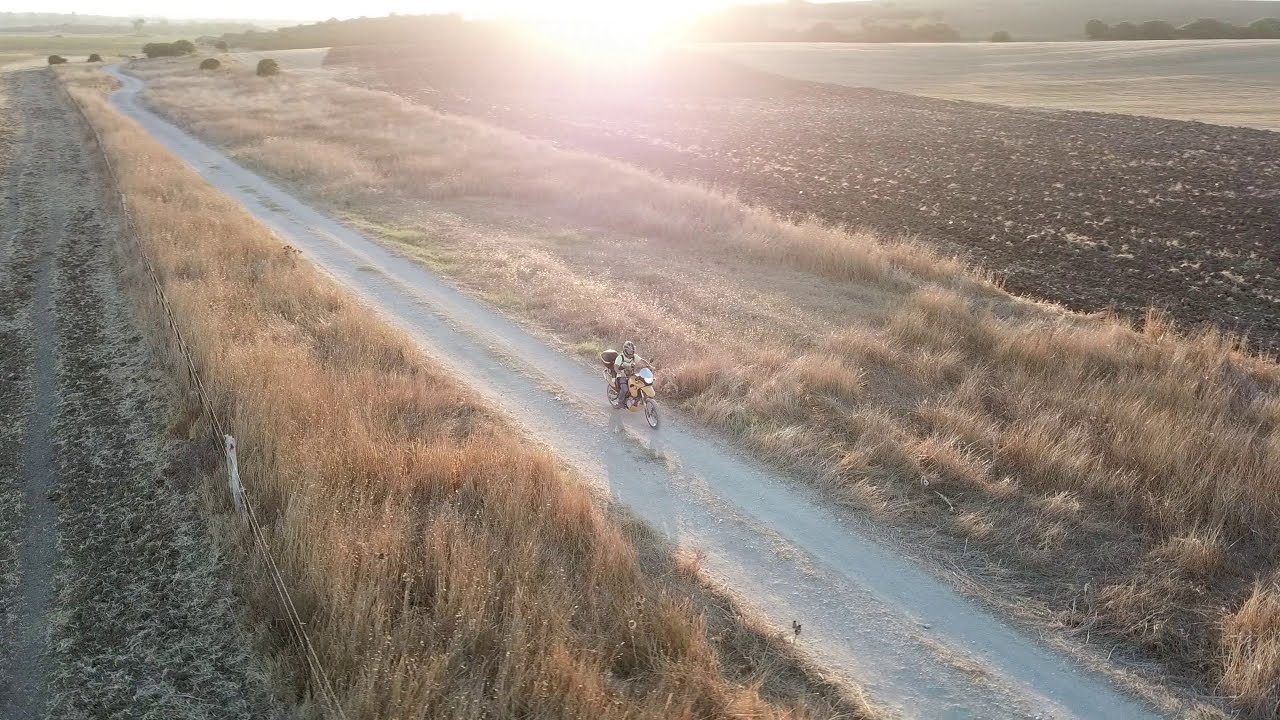The image captures a top-down view of a dirt road or trail stretching diagonally from the bottom center to the top left of the frame. At the center of the dirt trail, a lone rider is seen on what appears to be a light yellow motorcycle or dirt bike. The rider, dressed in jeans and a white t-shirt, wears a black helmet and has straps over their shoulders and chest for safety. The trail is flanked on both sides by long, dead grass or grain, adding to the desolate and rugged atmosphere. To the right of the trail, there's plain farmland extending into the horizon. On the left, a simple cord fence runs parallel to the road. The sun, positioned at the top of the image, casts a glaring light that covers about 10% of the frame, creating a beautiful yet harsh landscape.